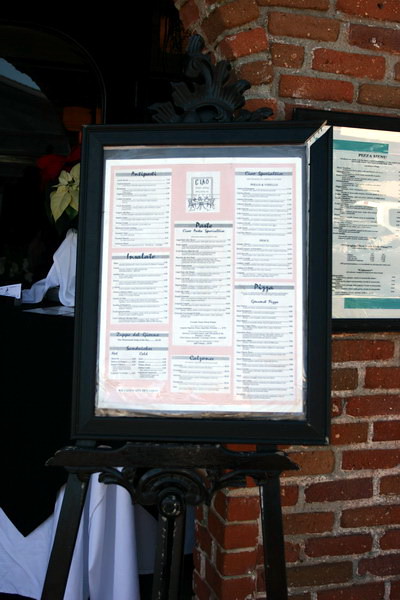In this horizontal photograph, the central focus is a menu showcased in a simple, thick, black wooden frame. The frame rests on a black easel, which is positioned in front of a brick wall. The menu itself is divided into three vertical columns, each set against a background of pink with white borders. At the top of each column are gray bars containing headings in large black script. Below these headings, rows of items are listed alongside numbers, suggesting that it is indeed a menu. 

In the background, there is an arrangement featuring a yellow flower placed atop a table with a white tablecloth and black draping. Additionally, another similar menu-like object is mounted under glass on the brick wall. The intricate details and layout of the image present a charming and meticulous display, indicative of a thoughtfully designed setting.